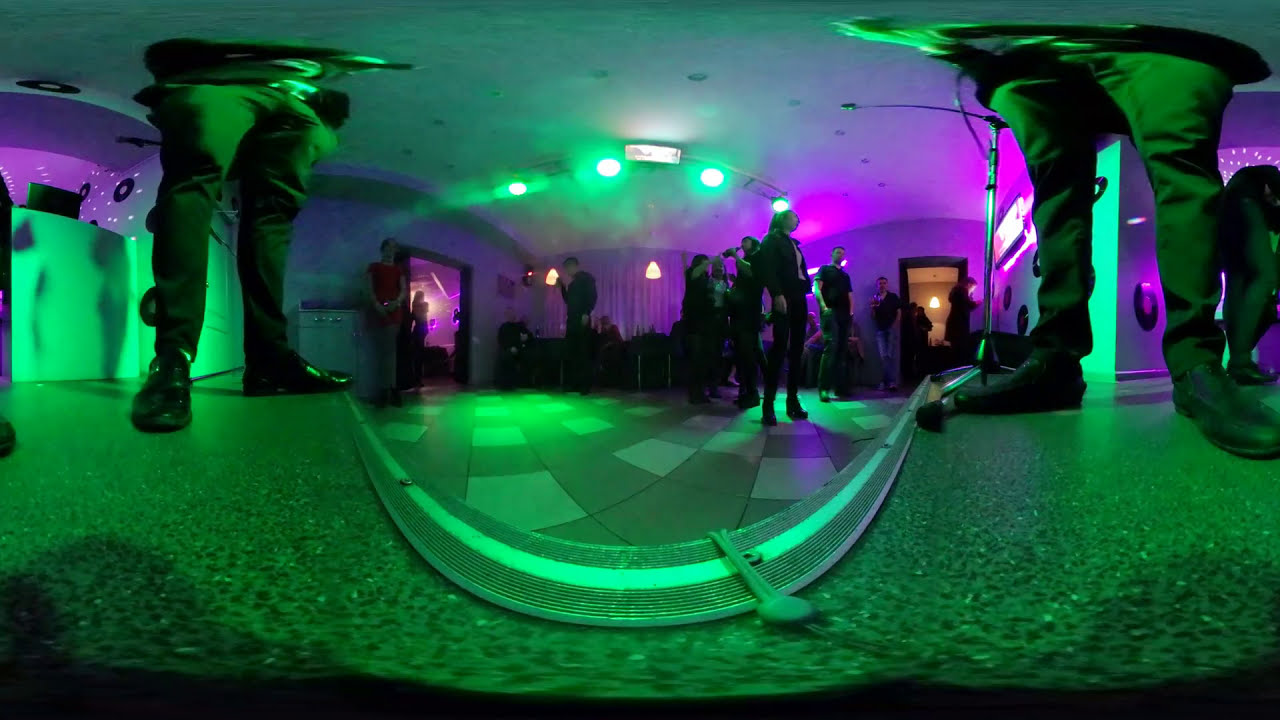The image portrays a distorted, 360-degree view of a small, intimate venue that could be a club or bar with a low white ceiling. At the forefront of the stage are the lower bodies of two men, likely musicians, dressed in black pants and black laced shoes, standing by microphones. The tiled floor, featuring a checkerboard pattern of white and brown tiles, extends outward into the room where several people are gathered, possibly audience members dressed in dark clothing. A silver, swooping arc with bands and a lever-like feature descends from the ceiling, contributing to the scene's distortion. The lighting above is composed of green and purple hues with stage lights shining onto the stage area, and round fixtures, perhaps lights, hang from the greenish ceiling. There are two doorways located at the left and right center of the room, suggesting access to other parts of the venue. The photo's overall green hue gradually transitions to purple, adding to its unique ambiance.